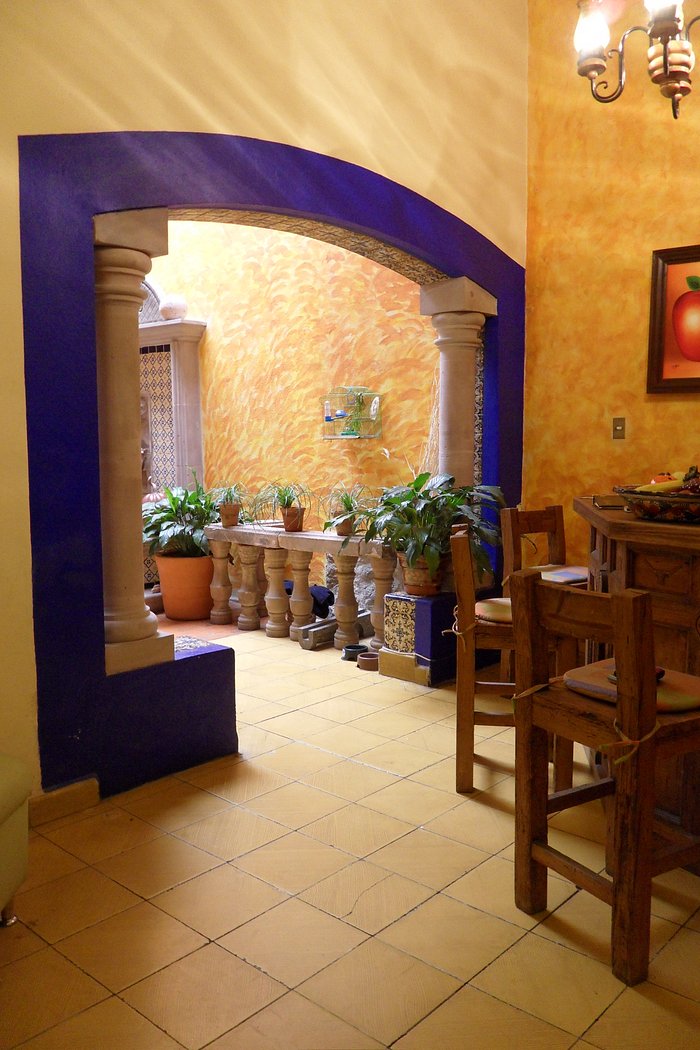The image depicts an indoor scene, possibly within a restaurant or a dining area of a stylish estate, featuring vivid Southwestern or Spanish interior design. The room is characterized by tall ceilings and walls adorned with a vibrant wave pattern in orange and yellow colors. The floor is made of orange tile. A striking blue archway with two white stone columns stands prominently, leading to another area filled with numerous potted plants, including three small ones atop the columns and a larger one on each end.

To the right, there's a sturdy wooden bar accompanied by high, rustic wooden stools, suggesting a breakfast bar or casual seating area. Above this space, a wooden chandelier can be seen illuminating the room. On the wall behind the bar, there's a partially visible painting, likely of an apple, adding a touch of artistry to the setting. An ornate print adorns the wall on the other side of the archway, enhancing the rich and intricate design of the space.